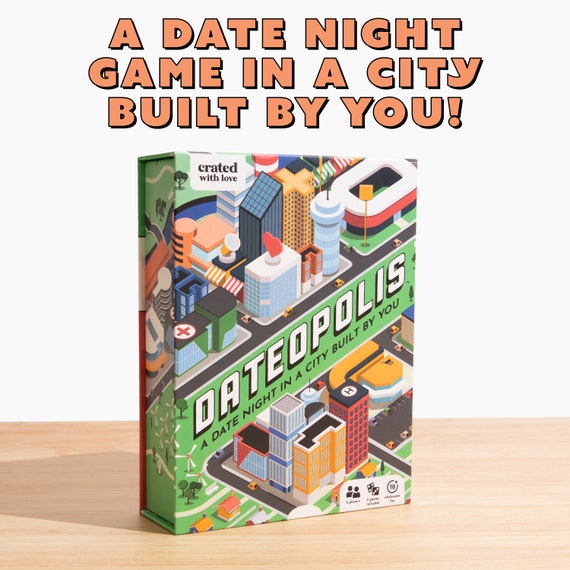This is an advertisement for Datopolis, a date night board game centered around building a city together. The eye-catching orange lettering at the top declares, "A date night game in a city built by you." The box, which is labeled with phrases like "Created with Love" and "Datopolis: A Date Night in a City Built by You," sits on a tan-brown wood grain surface. The white background underscores the box's colorful, cartoon-like cityscape design, reminiscent of The Sims, featuring skyscrapers, a helicopter landing port, roads, small buildings, windmills, a stadium, and a circular multi-story building. The overall scene is vibrant and inviting, capturing the essence of a playful and romantic evening.